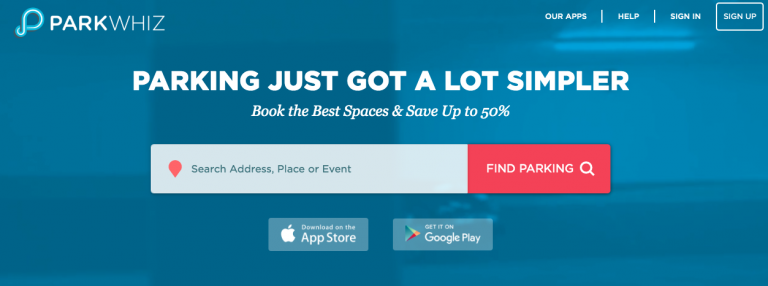This image depicts a promotional banner for a parking website, presented in a long horizontal format with a multi-shaded blue background that appears intentionally blurred. At the top left corner of the banner, the brand name "ParkWiz" is displayed alongside a small "P" icon. To the right of the brand name, there are links for "Our Apps," "Help," "Sign In," and a prominently outlined "Sign Up" button.

In bold white capital letters, the slogan "PARKING JUST GOT A LOT SIMPLER" dominates the center of the banner, with an italicized subheading below that reads, "Book the best spaces and save up to 50%." Beneath this tagline, a white search bar invites users to enter an address, place, or event to find parking. The search bar is complemented by an icon of an upside-down red teardrop, symbolizing a map pin, and placeholder text that says "Search address, place, or event." Attached to the search bar is a red button labeled "Find Parking," which includes a magnifying glass icon.

Towards the bottom of the banner, there are two rectangular buttons: one with the phrase "Download on the App Store" and another stating "Get it on Google Play," both encouraging users to download the ParkWiz mobile app.